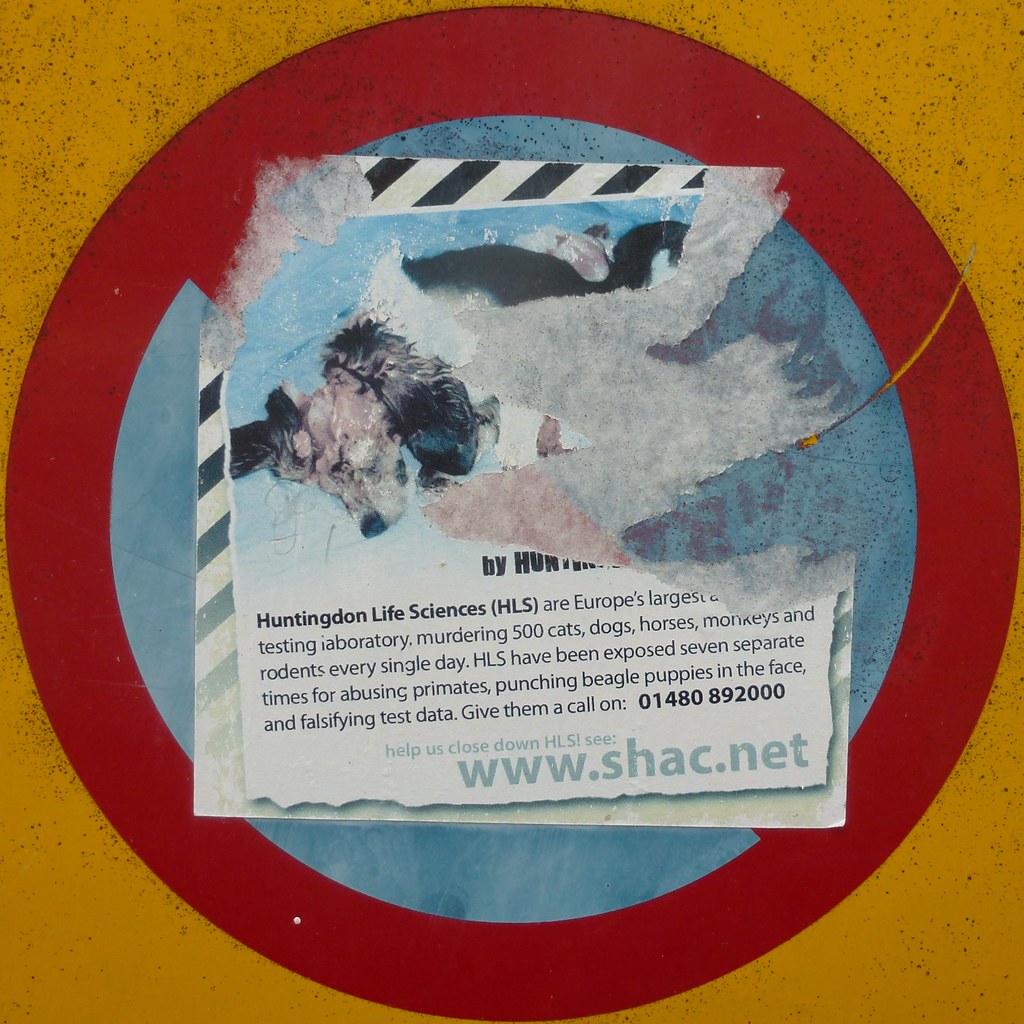Torn and partially obscured, an old protest poster is affixed to a yellow wall layered with faint black and gray speckles, reminiscent of a Magen painting. The wall features a wide red circle with a diagonal red slash from top left to bottom right, suggesting prohibition. Inside this circle are two blue hemispheres, partially obscured by the torn poster. The white poster itself bears black lettering reading "Huntingdon Life Sciences (HLS)" with parts of it ripped away. Visible text includes bleak statements about HLS being "Europe's largest testing laboratory," "murdering 500 cats, dogs, horses, monkeys, and rodents every single day," and detailing abuse such as "punching beagle puppies in the face and falsifying test data." The bottom of the poster includes a call to action in light blue text, directing viewers to "www.shac.net" to support the closure of HLS. The poster's edges are tattered, revealing glimpses of the underlying anti-action symbols and adding to the sense of urgency and outrage conveyed by the messages.